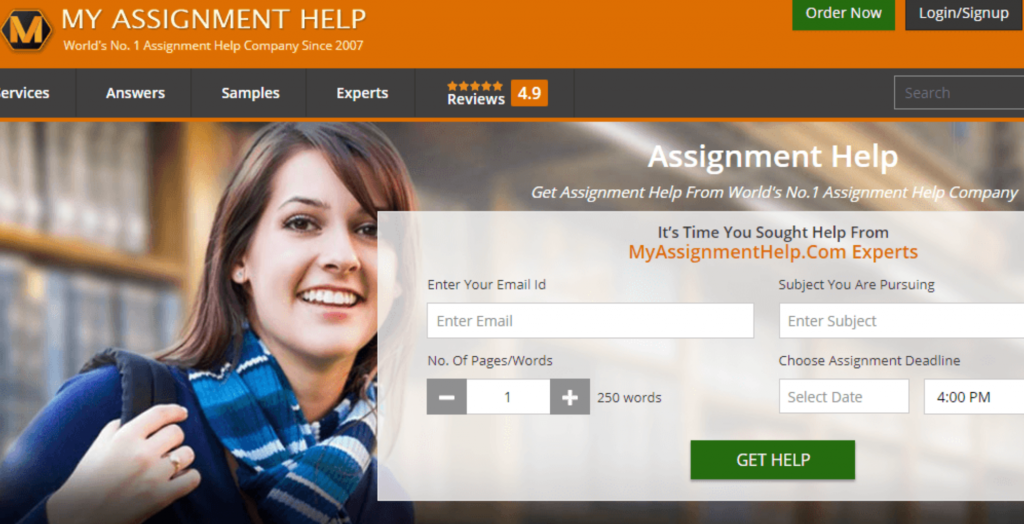The banner at the top of the image prominently features an orange strip with the text "World's Number One Assignment Help Company Since 2007" on the left side. On the right side of this strip, there is a green "Order Now" button with white font, and next to it, a black "Log In/Sign Up" button with white font. Below this strip is a dark slate gray or black section featuring navigation items in white font: from left to right, these are "Services" (though the 'S' is partially cut off), "Answers," "Samples," "Experts," "Reviews," and a "4.9" rating. To the far right, there is a search bar, which is also partially cut off.

The main section below this contains an image of a young Caucasian woman with dark hair, wearing a blue long-sleeve shirt and a blue striped scarf around her neck. She has a backpack slung over her right shoulder. Next to her, text offers the promise "Assignment Help" followed by "Get assignment help from the world's number one assignment help company. It's time you sought help from myassignmenthelp.com experts." Below this text is a form with a search field labeled "Enter your e-mail ID," which seems odd in context. To the right of this field, another labeled "Subject You Are Pursuing" asks the user to "Enter Subject" in a designated data field. Directly beneath these fields is a section that requests the "Number of Pages/Words," pre-populated with the number one in the field, flanked by plus and minus buttons for adjustment.